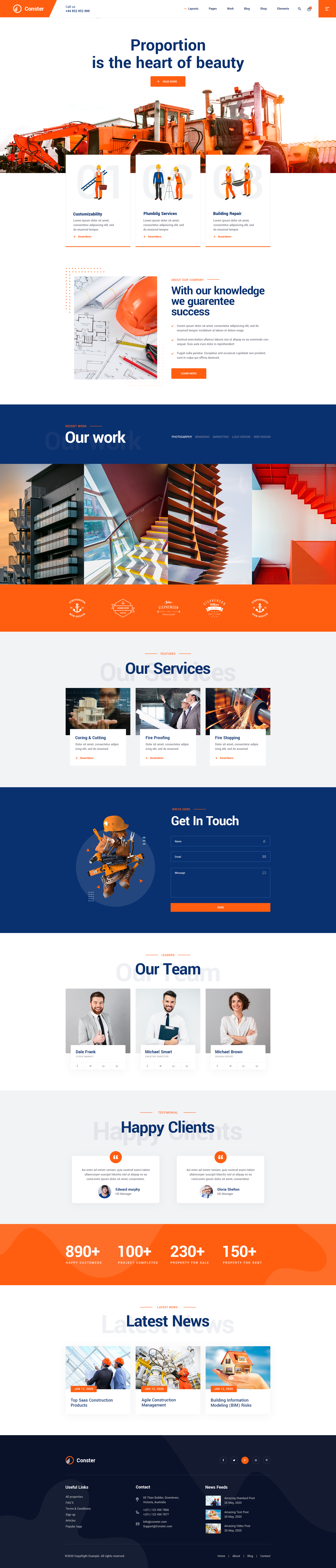This image captures the detailed layout of a web page for "CONSTR" (C-O-N-S-T-R).

At the top of the page, the navigation menu includes links to Layouts, Pages, Work, Blog, Shops, Elements, a search box, and a shopping cart icon. Below the menu bar, a prominent heading states, "Proportion is the heart of beauty," accompanied by an orange "Read More" button and a photo featuring various orange tractor trucks.

Following this, three clipart images represent different services labeled Customizability, Plum Egg Services, and Building Repair, with accompanying descriptions in an unknown language. 

The next section is titled "About Our Company" with the statement, "With our knowledge, we guarantee success," and a visual to the left depicting a hardhat, a blueprint, measuring tape, and a pencil, symbolizing workplace tools.

The "Recent Work" section showcases clickable categories such as Photography, Branding, Marketing, Logo Design, and Web Design, with relevant images displayed below each category. Following this, logos all labeled "John Stevenson" in white against an orange background appear, showcasing various logo designs.

The "Features, Our Services" section lists three core services: Curring and Cutting, Fireproofing, and Firestopping, each followed by descriptions in another language.

A "Get In Touch With Us" section encourages visitors to contact the company, featuring fields for name, email, and a message, along with a "Send" button. Above this, there’s text reading "WRITEHER."

The "Our Team" section presents three team members: Dale Frank (Start Market), Michael Smart (Creative Director), and Michael Brown (Design Expert), each with social media links for Facebook, Twitter, Google, and LinkedIn.

In the "Testimonials" section, a large logo reads "Happy Clients" in blue, followed by testimonials from Edward Murphy and Gloria Shelton, both HD Managers, with their content in a different language.

An "Advertising" section highlights the company's accomplishments, including "890+ Happy Customers," "100+ Projects Completed," "230 Property for Sale," and "150+ Property for Rent."

The "Latest News" section features three posts dated January 12, 2020:
1. "Top SAAS Construction Products" - Image of two men with hard hats examining a project.
2. "Agile Construction Management" - Relevant themed image.
3. "Building Information Modeling (BMI)" - Picture of a small house in a hand.

Finally, the footer section includes the site name "CONSTR," useful links, contact information, and news feeds.